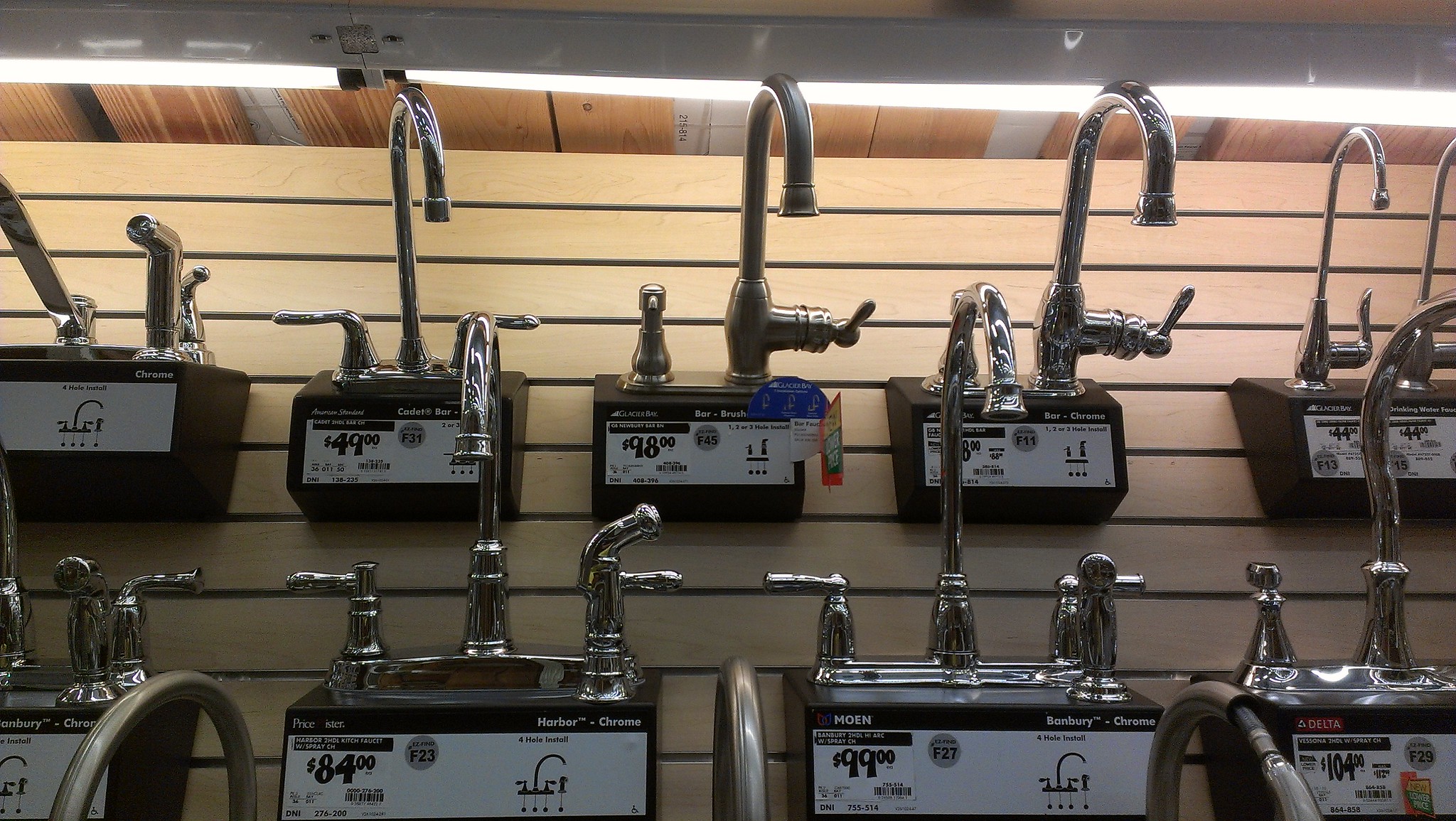This photograph, taken inside a hardware store, showcases an in-store display of various types of silver, stainless steel faucets arranged in two rows against a distinctive light brown wooden backdrop. At the upper part of the image, there is a white horizontal metal piece adorned with attached illuminating lights, casting a bright light over the display, with the store's ceiling featuring several vertically-oriented, light brown wooden slats. 

The faucets, varying in design from tall and thin to thick and compact, with some featuring an additional sprayer, are mounted on a shelf-like structure made of horizontal wood panels. 

Each faucet has a corresponding price tag on a white background below it, detailing the cost and, in some instances, the brand and finish type. Specific prices visible include $44.99, $48, $84, $98, $99, and $104. Notably, one faucet branded as Moon, with a chrome finish, is priced at $99. The display provides shoppers with clear information and easy access to various faucet options, enhancing their in-store buying experience.